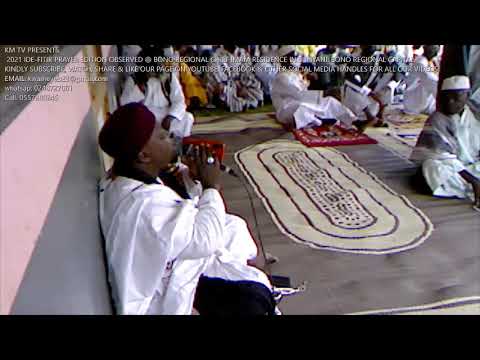The image depicts a communal gathering, possibly inside a mosque or a similar religious or cultural setting. The focal point is a dark-skinned man positioned slightly left of center, leaning against a gray and pink wall, and holding a microphone in his right hand, which is adorned with a large ring. He is speaking to a group of people wearing long white robes and round caps of various colors, who are seated cross-legged on patterned rugs with distinctive oval-shaped borders in the middle of the room. Overhead, a text banner reads "KMTV presents 2021 IDE... prayer," though the small font makes the full text difficult to decipher. The image is framed by black bands at the top and bottom, and the main colors in the scene are brown, gray, white, with some pink accents.